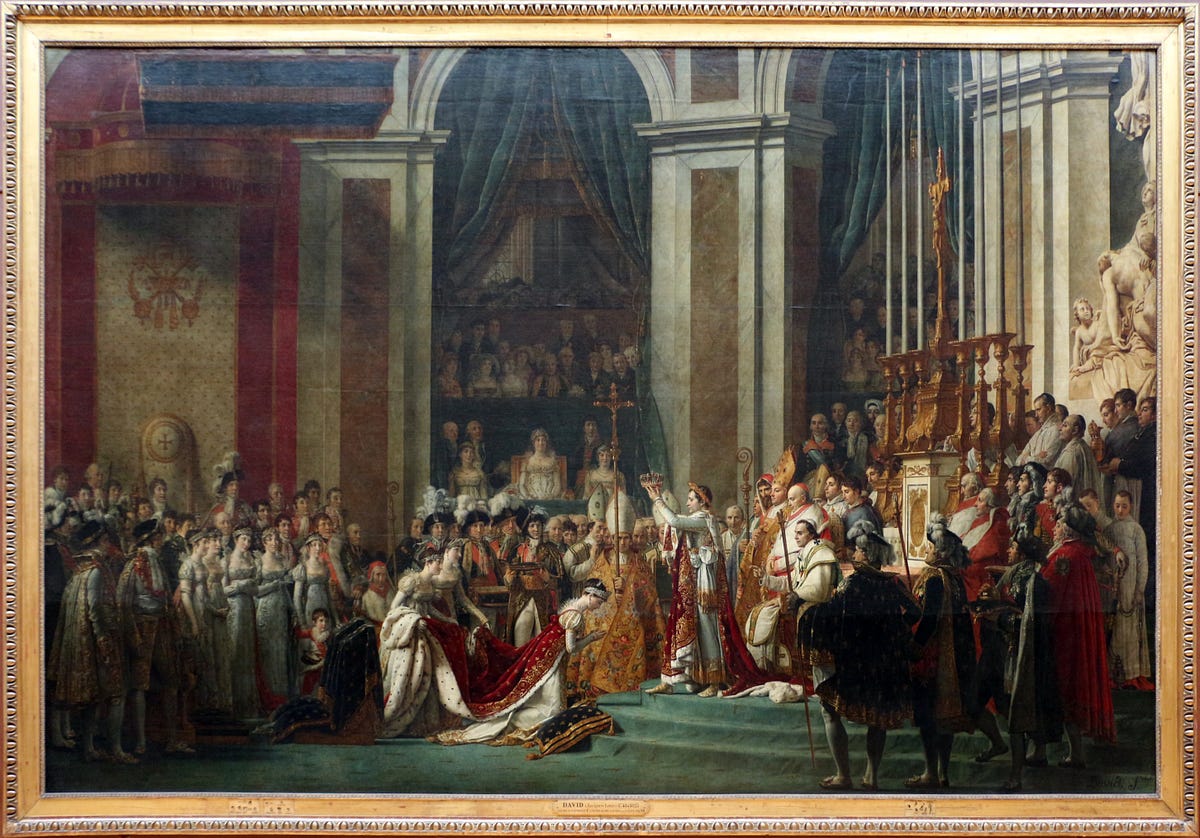This high-quality landscape oil painting, framed by an ornate gold edge with dark blue embossed details, captures an elaborate medieval court scene set within a chapel-like interior. The composition centers around the knightly crowning of what appears to be a princess or queen, dressed in a white gown with a red velvet cloak adorned with gold accents. She kneels on pillows, hands in a praying position, as a man in a similarly opulent red velvet cape stands a few stairs above her, poised to place a crown upon her head. Surrounding them are men and women in elaborate traditional attire—men draped in capes and women in long, elegant dresses, some with headbands. The scene is rich with details: a priest holds a large cross, tall candlesticks illuminate the background, and ornate sculptures—including one depicting Jesus on the cross—adorn the altar. The backdrop features two white arches with brown vertical stripes and a red doorframe with gold banding on the left. The painting exudes grandeur and reverence, highlighting the ceremonial splendor of the medieval era.